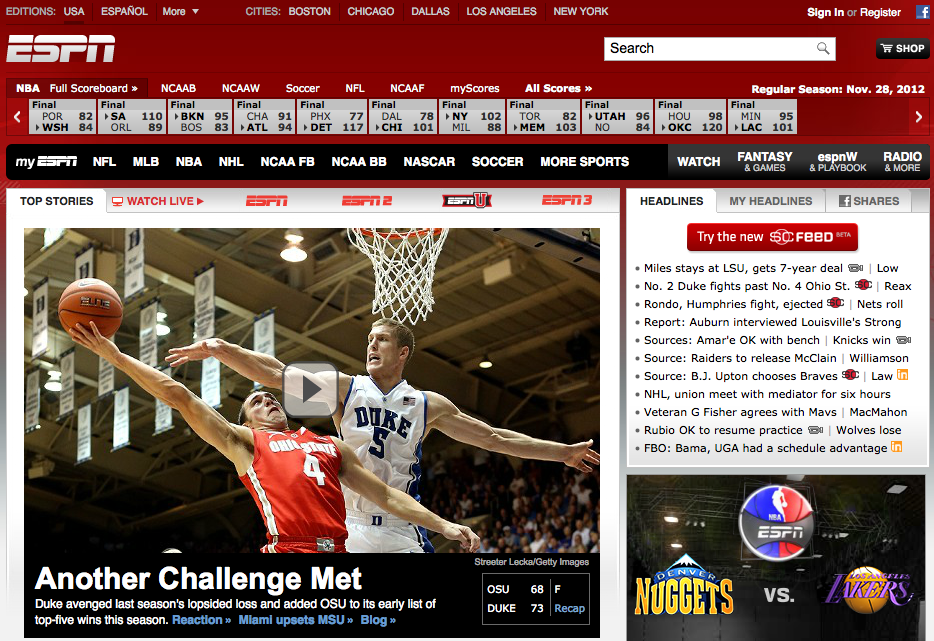The ESPN homepage screenshot showcases a well-organized sports news portal with various features for easy navigation and information retrieval. 

At the very top left, the familiar white ESPN logo stands out, above which is a section offering different editions like USA and Español, alongside city-specific editions including Boston, Chicago, Dallas, Los Angeles, and New York. To the top right, users can find options to "Sign In" or "Register" and a blue and white Facebook logo for social media connectivity.

Central to the page, a prominent ESPN banner is displayed. To the center right, there's a conspicuous search bar in white with black text, and next to it, a black button with a white shopping cart silhouette labeled "Shop."

Directly below, there's a live scores section with the NBA scores highlighted, displaying around ten recent final scores. Other tabs available but not open include NCAAB, NCAAW, Soccer, NFL, NCAAF, "My Scores," and "All Scores." The regular season date is noted as November 28, 2012.

Below the scores, there's a broader sports navigation section covering NFL, MLB, NBA, NHL, Soccer, and others like NASCAR. Below this, a prominent photograph serves as a thumbnail for a video. The image captures an intense moment from a college basketball game between Ohio State and Duke. The Ohio State player in a red jersey is in action, attempting a shot, while a Duke defender in a white jersey is poised to block it. The scene is set in Duke's stadium with visible white hoops and rafter banners. Captioned below the image: "Another challenge met. Duke avenged last season's lopsided loss and added OSU to its early list of top five wins this season." Highlighted in blue nearby is a link stating "Reaction: Miami upsets MSU" and "Blog."

Adjacent to this image is the game's final score: OSU 68, Duke 73. Below this information is a section with multiple sports headlines, approximately ten, along with a red button inviting users to "Try the new SC feed." At the bottom right of this segment, you see logos for the Denver Nuggets versus the Los Angeles Lakers, and centrally, at the top, there's an NBA ESPN logo in red and green.

This detailed snapshot provides a rich overview of the ESPN homepage layout, focusing on its broad array of sports content and user-friendly features.